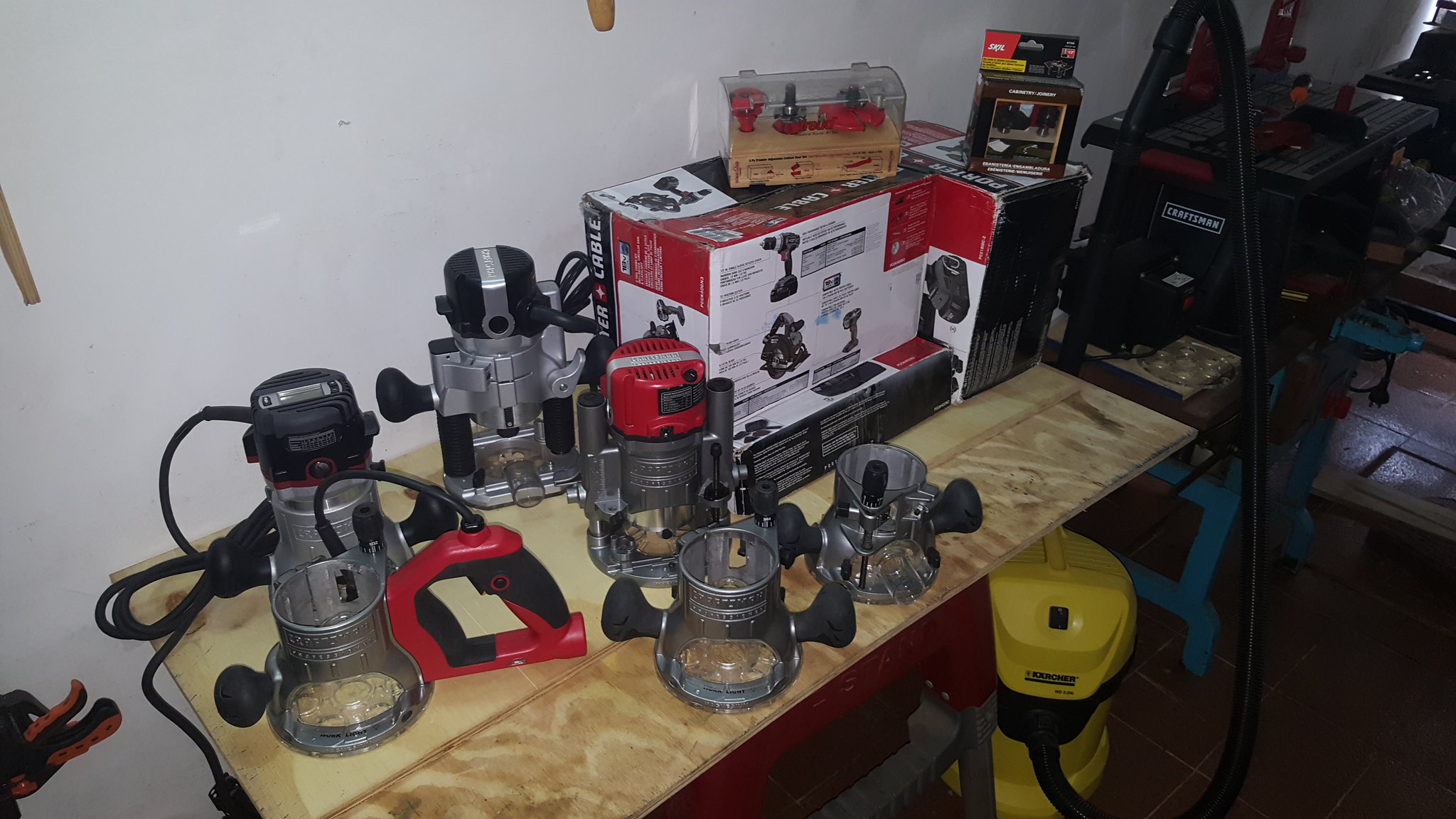The photograph reveals a cluttered workshop or garage setting with a white wall serving as the backdrop. Dominating the scene is a wooden table crafted from a piece of plywood, upon which a variety of tools and boxes are scattered. Underneath the table, a yellow canister-style shop vacuum with a long extension hose is prominently visible. Adjacent to it lies a Craftsman saw. On the tabletop, there are several boxes, some assumed to contain cordless drills and saws, and additional tools or attachments stacked on top of them. 

In the foreground, a metallic cup with a transparent section near the bottom is attached to a red and black handle with a black power cord extending from it. Nearby, two identical cups without handles are positioned, with three more similar cups towards the back, each holding motor-like devices featuring black tops, indicative of electrical components such as sanders or small wood shapers. The assortment of tools, including unidentified silver and black devices with power cords, hints at an extensive and busy workspace designed for various electronic and manual tasks.